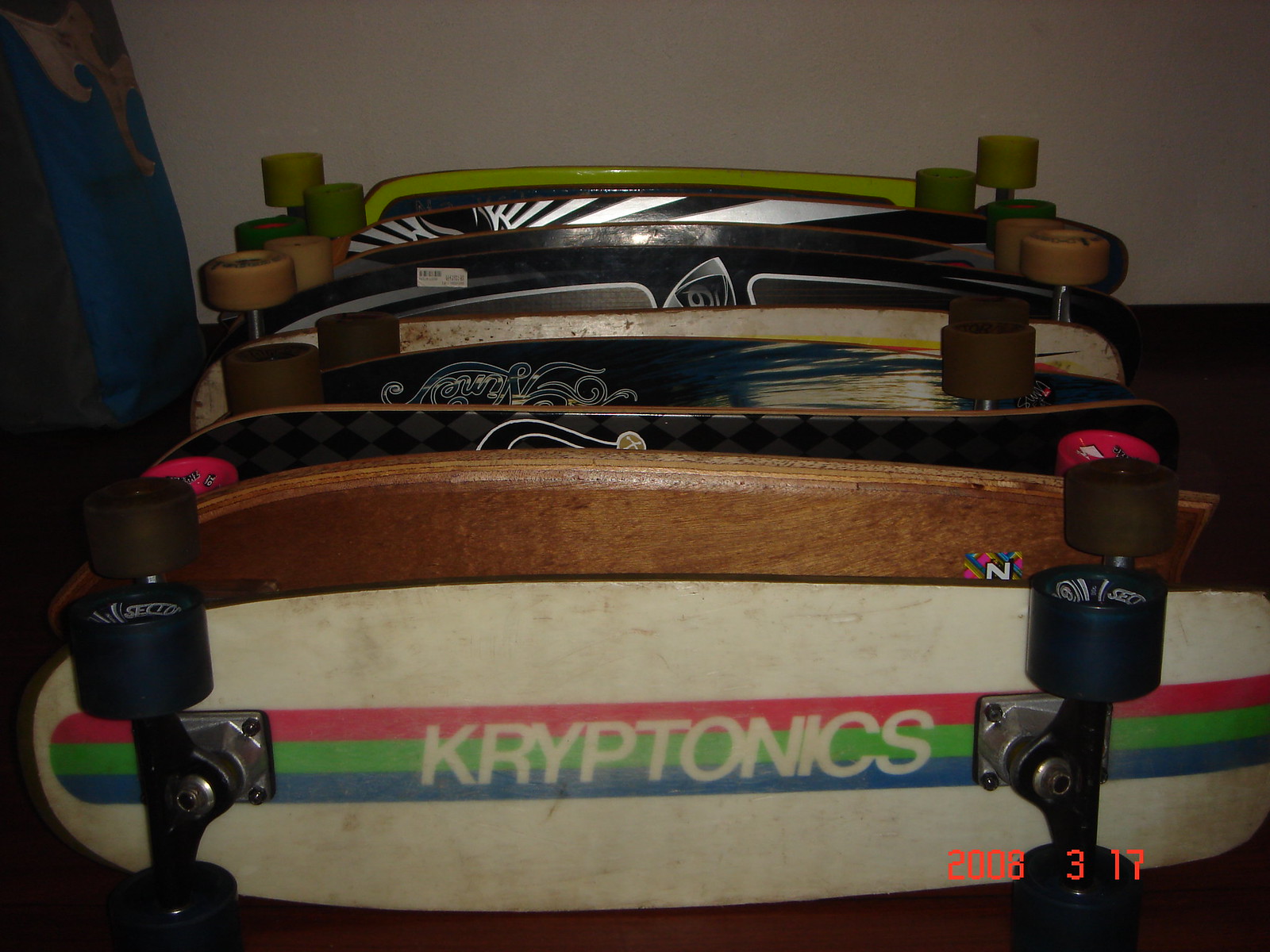The image is a color photograph taken in landscape orientation, featuring a row of skateboards lined up on their sides, one behind the other, stretching back into the distance. In the bottom right corner, there's an orange date stamp from an old-school 35mm camera, marking the date as March 17, 2008. 

The skateboard closest to the viewer is prominently displayed with its bottom facing forward. This skateboard features the brand name "Kryptonix" inscribed horizontally along its length, accompanied by three colored stripes—reddish-pink, green, and blue. It has black wheels, distinctly standing out from the others. 

Behind the front skateboard, there are several others visible in the line-up. Although the details become less clear moving backward, the immediately following skateboard appears to be a dark oak wood. Further back, patterns and colors emerge, including a black and gray checkerboard design and a bright green skateboard at the very end of the line. Various other boards intermingle with colors and graphics, some showing signs of wear. The wheels among the skateboards vary, including brown, beige, and green tones.